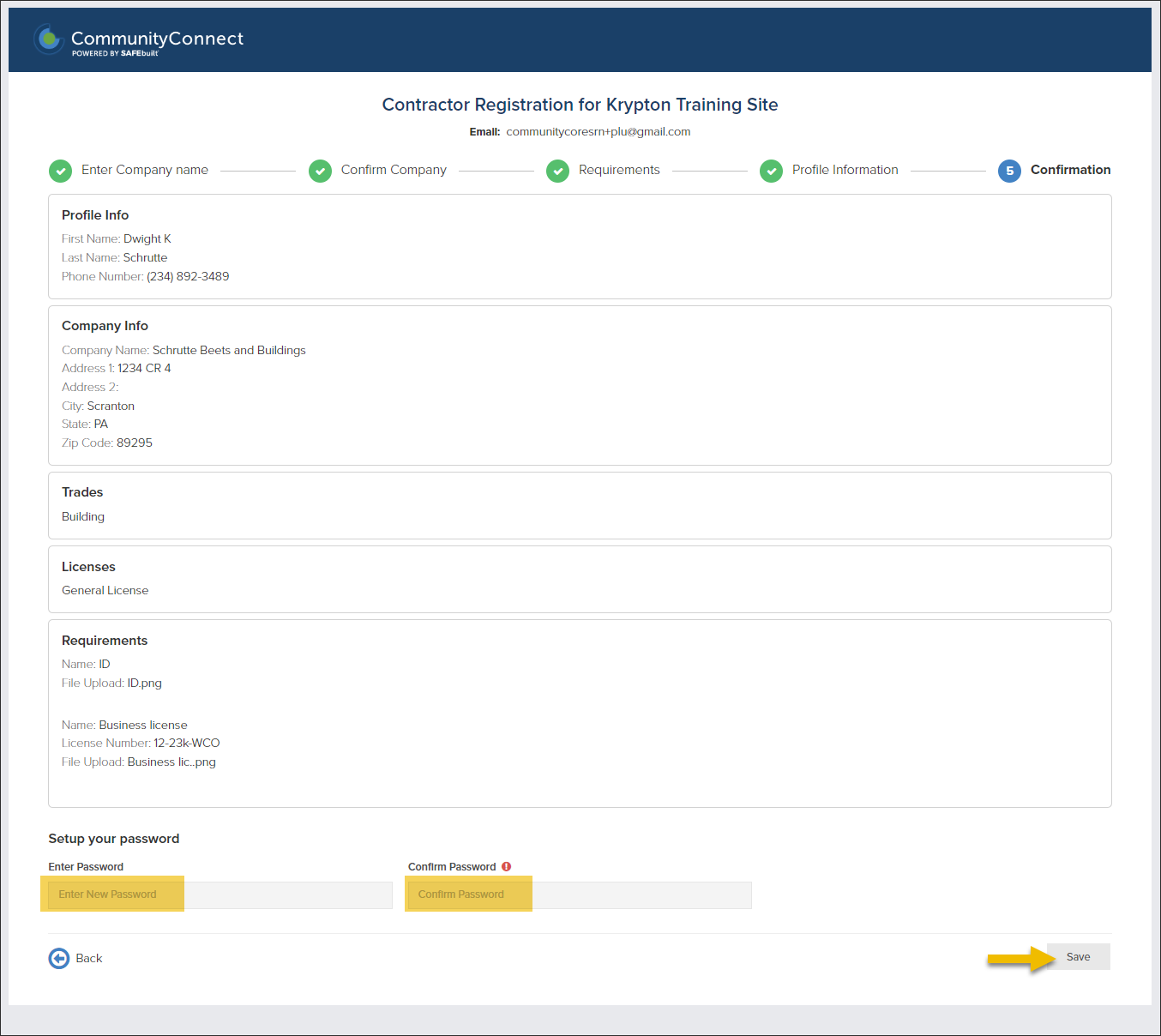**Detailed and Cleaned-Up Caption:**

This image is a screenshot of a web page designed for contractor registration on the Krypton Training Site. At the top, there is a blue banner featuring a white logo on the left side that reads "Community Connect," and beneath it, smaller text that says "Powered by SafeBuild." 

Below this blue banner, the background shifts to white. Centered at the top in bold blue text is the title "Contractor Registration for Krypton Training Site." Following that, in smaller black text, it reads "Email Community Chorusin plus PLU at gmail.com."

The main body of the page shows several steps indicated by green check marks, each with corresponding text: "Enter company name," "Confirm company requirements," and "Profile information." These steps span across the width of the page. Next, there is a blue circle with a white number five inside it, followed by black text reading "Confirmation."

Further down, there is a section labeled "Profile Info." It includes form fields with the following details: 
- First Name: Dwight K
- Last Name: Chirrut
- Phone Number: 234-892-3489

Under "Company Info," the details are:
- Company Name: Chirrut Beets and Buildings
- Address Line 1: 11234 CR 4
- Address Line 2: (blank)
- City: Scranton
- State: PA
- Zip Code: 89295

For "Trades," it lists "Building" and, under "Licenses," it has:
- General License: License number 12-23K-WCO

In the "Requirements" section, it includes:
- Name: ID
  - File Upload: ID.png
- Name: Business License
  - License Number: 12-23K-WCO
  - File Upload: businesslice.png

Towards the bottom, there is a section to "Set Up Password," highlighted in yellow. This section includes boxes to enter and confirm the password. Finally, in the bottom right corner, there is a "Save" button with a yellow arrow pointing towards it.